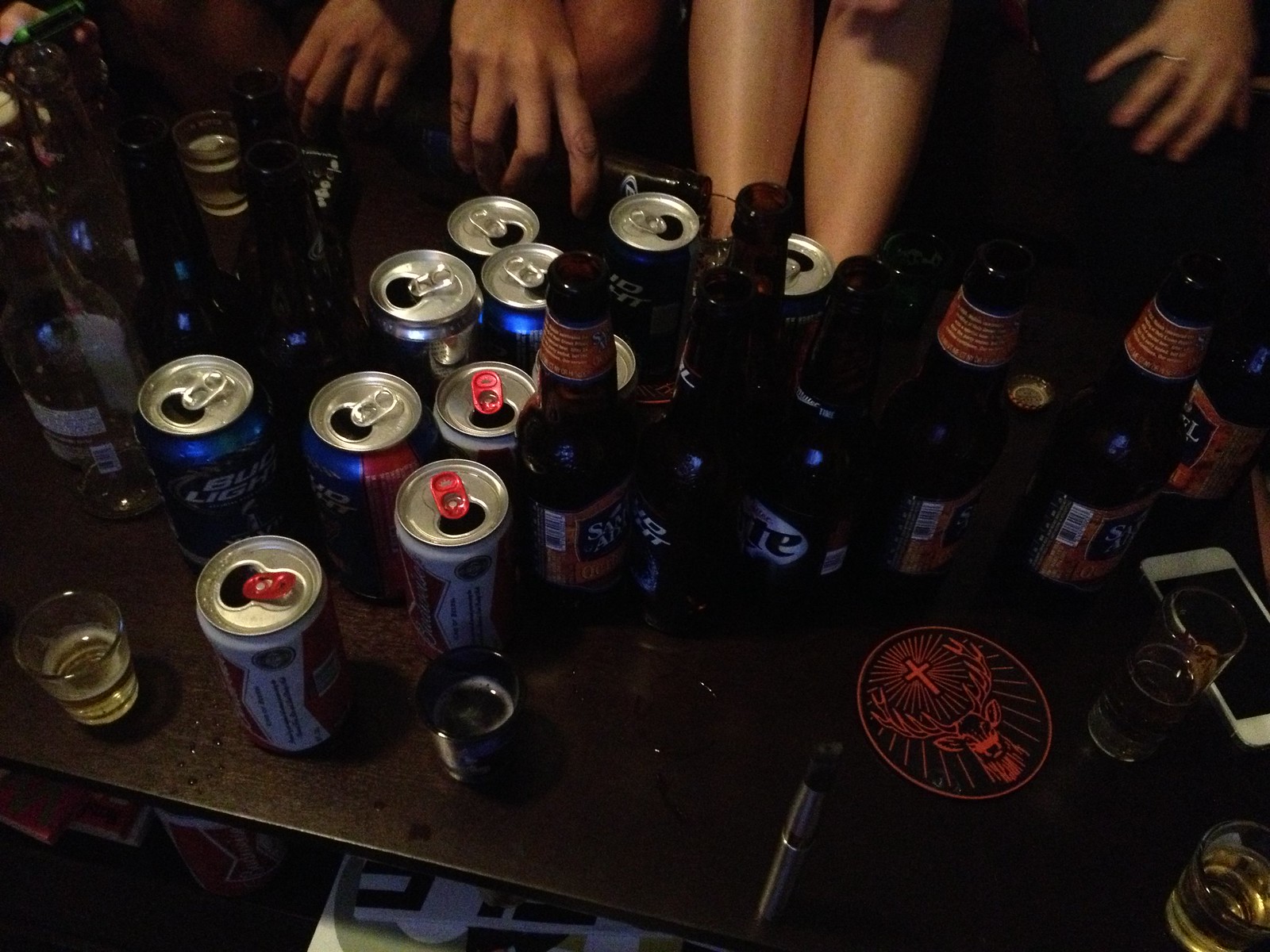The photograph, taken indoors at night, captures the aftermath of what appears to be a college party. The central focus is a dark brown wooden table cluttered with empty beer bottles and cans, including identifiable brands like Bud Light, Sam Adams, and Miller Lite. Among the scattered items are glasses containing a golden substance, possibly whisky, and a shot glass. An iPhone lies face up on the bottom right corner of the table. Underneath the table, cases of beer are visible along with a white item featuring a grey logo. A Jägermeister coaster with a red stag and cross logo stands out on the table. In the background, dimly lit hands and legs of at least three individuals are visible, suggesting the presence of people who have yet to tidy up from the night’s festivities.